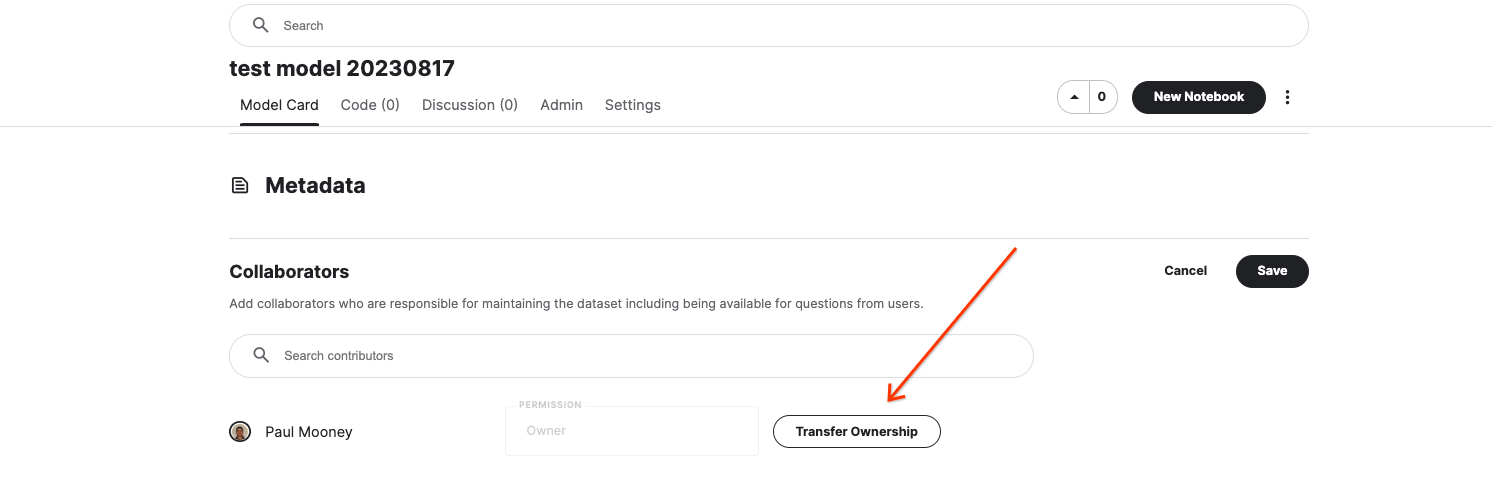A minimalistic search interface is depicted, tailored for dataset management rather than car searches. The user has input a search term and the results displayed include a test model labeled "202-308-17". There is minimal accompanying information. Metadata is mentioned, with a prompt to add collaborators responsible for maintaining the dataset. 

Toward the bottom of the interface, one item is listed with the name "Paul Mooney" identified as the permission owner. Next to this, there is a "Transfer Ownership" button, which is highlighted by a red arrow, suggesting a function to reassign dataset responsibility from Paul to another user.

At the top right corner, the interface features a black "New Notebook" button and a "Save" button. Additional navigation tabs labeled "Admin" and "Settings" are also visible, indicating further administrative options for managing the dataset.